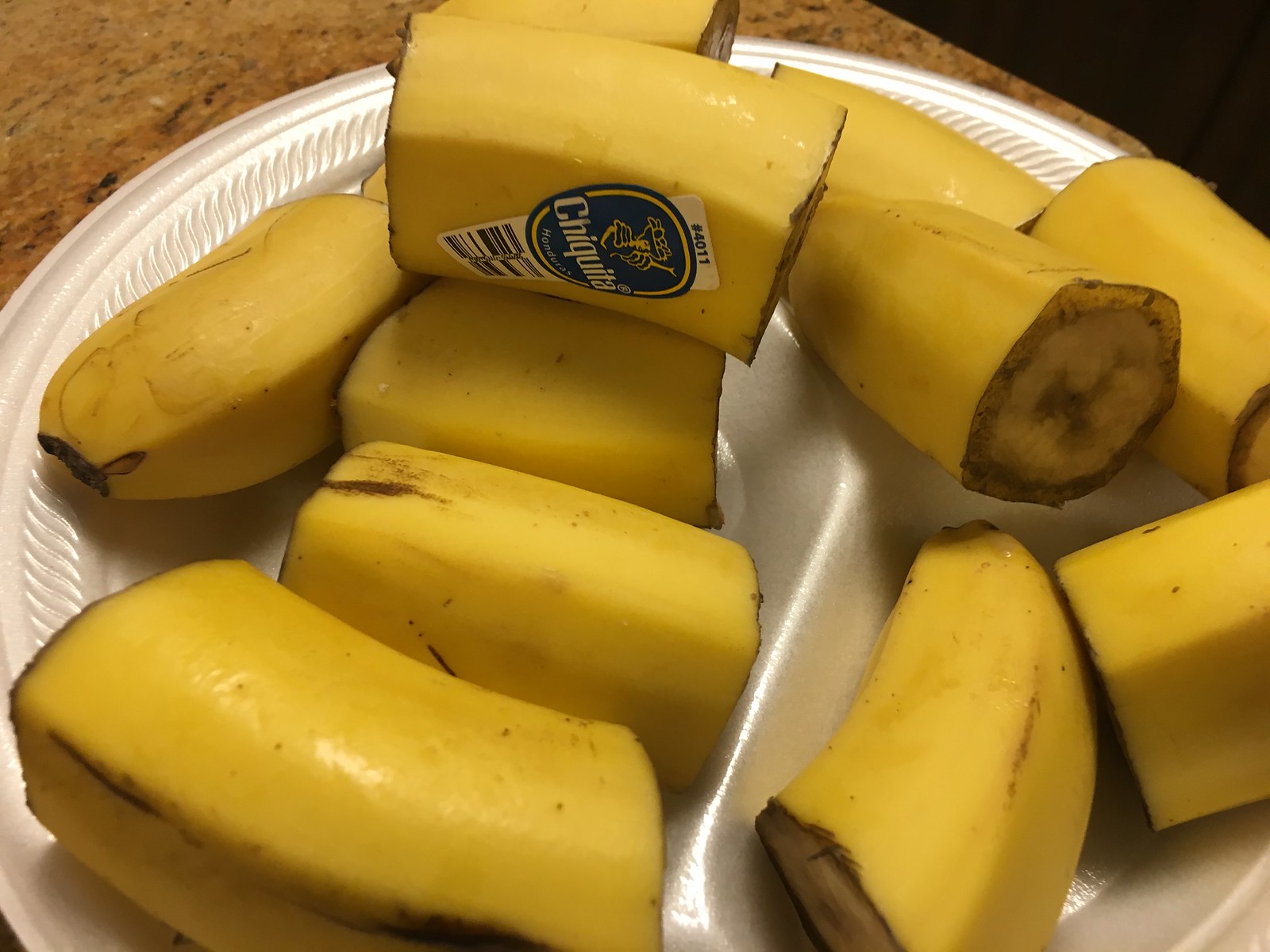This color landscape photograph features sliced Chiquita bananas with their peels intact, arranged on a disposable, off-white, styrofoam plate divided into compartments. The bananas, varying in ripeness and showing some browning on the edges, are cut into approximately two-inch segments and piled onto the plate. A piece positioned near the top center prominently displays the Chiquita label, number 4011, and a barcode. The plate rests on a granite countertop with shades of brown, adding depth to the setting.